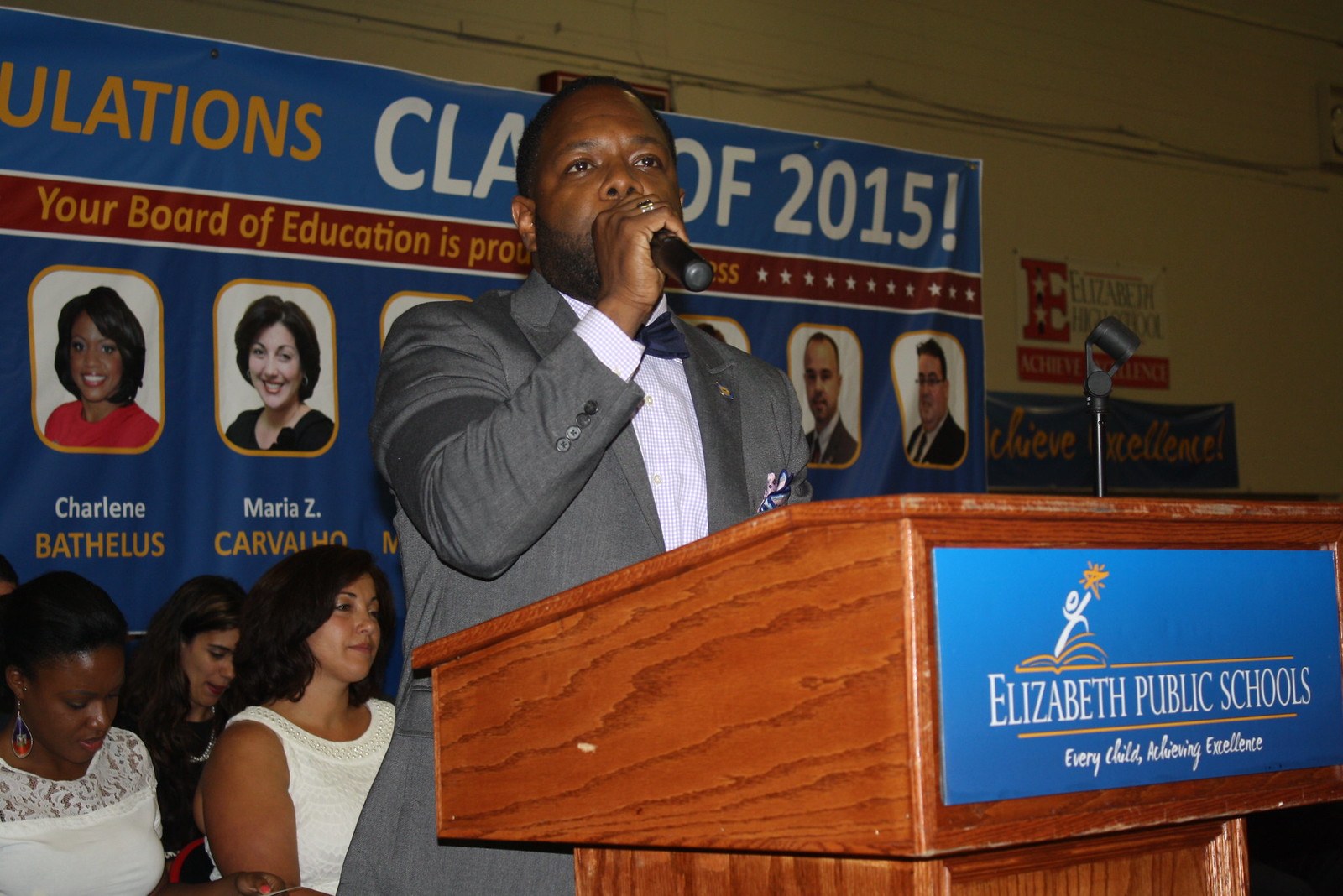In this photograph, a distinguished black man, characterized by his short black hair and black beard, stands at a wooden podium with a microphone raised to his mouth. He is confidently grasping the microphone with one hand, as he addresses the audience with a solemn expression. He is attired in a light gray blazer over a plaid collared shirt that blends light purple and dark blue hues, complemented by a dark blue bow tie partially obscured by his hand. The podium, made of light orange wood with visible chips, prominently features a blue plaque with white text that reads "Elizabeth Public Schools" and underneath, "Every Child Achieving Excellence." An emblem depicting a white stick figure jumping out of a yellow book and reaching for a yellow star accompanies the text.

Behind the speaker, seated to his left, are three women, each providing further context to the image. To the front left, a black woman in a white dress looks downwards, while a Hispanic woman with shoulder-length black hair in an identical white dress gazes ahead. Positioned slightly back, a third woman, possibly Caucasian or Hispanic, with black hair streaked with blonde and wearing a partially obscured black dress, sits further behind.

In the background, a shadowed cream-colored wall frames a large banner adorned with photographs and partially obscured text. The visible sections of the banner proudly announce, "Congratulations Class of 2015," and include portions of a message from the Board of Education, along with names such as Charlene Bathalis and Maria Z. Carvalho. This celebratory backdrop, featuring images of board members, hints at a formal, likely graduation event where achievements are being celebrated.